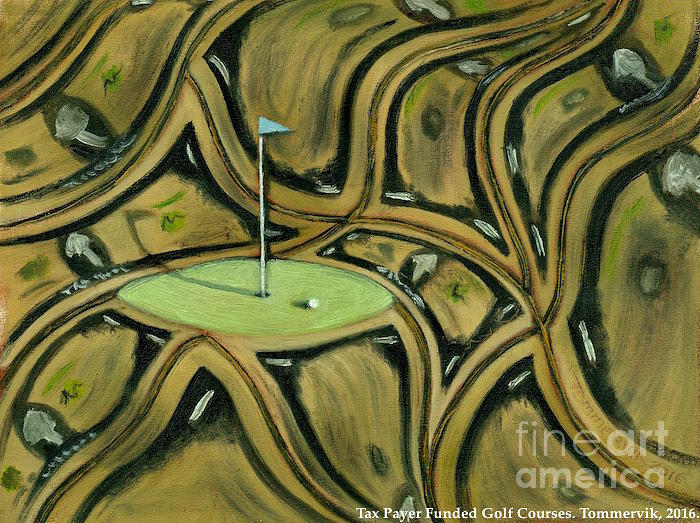This image is a fine art painting depicting a somewhat abstract representation of a golf course. Dominated by hues of greens, yellows, and beiges with splashes of black and white, the composition centers around a circular green area representing a golf green. On this green, a white flag stick with a blue triangular flag flutters, casting a shadow to the left. Adjacent to the flag stick, a white golf ball lies on the green. Surrounding the green, there are intricate, almost street-like shapes, resembling little roads coursing through the golf course, tinged in yellow and tan with white blotches. The background is a blend of brownish-green hues creating a complex, multi-directional roadway design. In the lower right corner of the painting, white lettering reads "Fine Art America, Taxpayer Funded Golf Courses, Tomervick 2016."